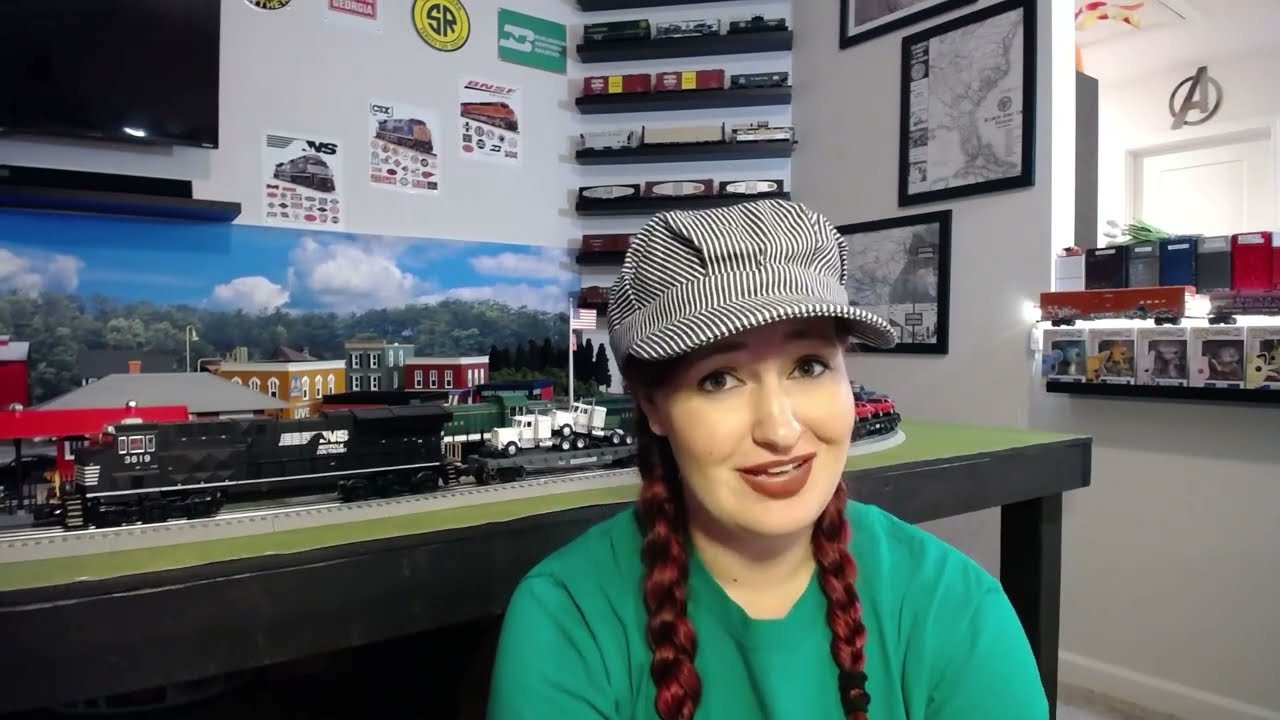The image features a woman with light skin and reddish-purplish braids that cascade down to her chest, adorned in a light green short-sleeved shirt. She sports a black and white striped train conductor's hat, its bill casting a slight shadow over her eyes. Her lips are painted red, and she appears to be seated, possibly on the ground or a small chair, while looking directly at the camera with an expression as if she’s speaking.

Behind her is a vibrant model train setup atop a green and black table. The train set includes a large black engine, pulling carts that carry white semi-truck cabs. The scene is surrounded by miniature buildings set against a backdrop of green hills and a blue sky scattered with clouds. The surrounding walls are adorned with various railroad-themed décor, including little framed posters, art pieces, and numerous train models displayed on black shelving units. To her right, under a window, additional rail models are visible, alongside a stack of pop toys. A TV is mounted on the wall in one corner, and a silver Marvel Avengers logo is seen above a distant door, completing the eclectic room's ambiance.